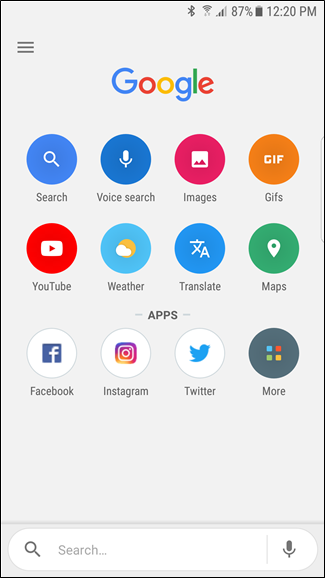The image features a smartphone interface against a gray background. In the upper right corner, there are icons indicating Bluetooth connectivity with three out of four bars, an 87% battery level, and the time shown as 12:20 PM. Below these icons is the Google logo, followed by a grid of 12 oval-shaped icons arranged in three rows of four.

- **Top Row:**
  - The first icon on the top left has a blue background with a white magnifying glass labeled "Search".
  - To its right, the next icon is a darker blue oval featuring a white microphone labeled "Voice Search".
  - The third icon has a red background with a photo icon labeled "Images".
  - The fourth icon in this row is an orange oval labeled "GIFs" with large white letters spelling "GIF".

- **Second Row:**
  - The first icon on the left has the YouTube logo.
  - Next to it on the right is a blue icon with a sun and cloud symbol, labeled "Weather".
  - The third icon in this row is for the Google Translate app.

The arrangement and details of each icon make it easy to navigate the Google interface, providing quick access to various Google services and utilities.